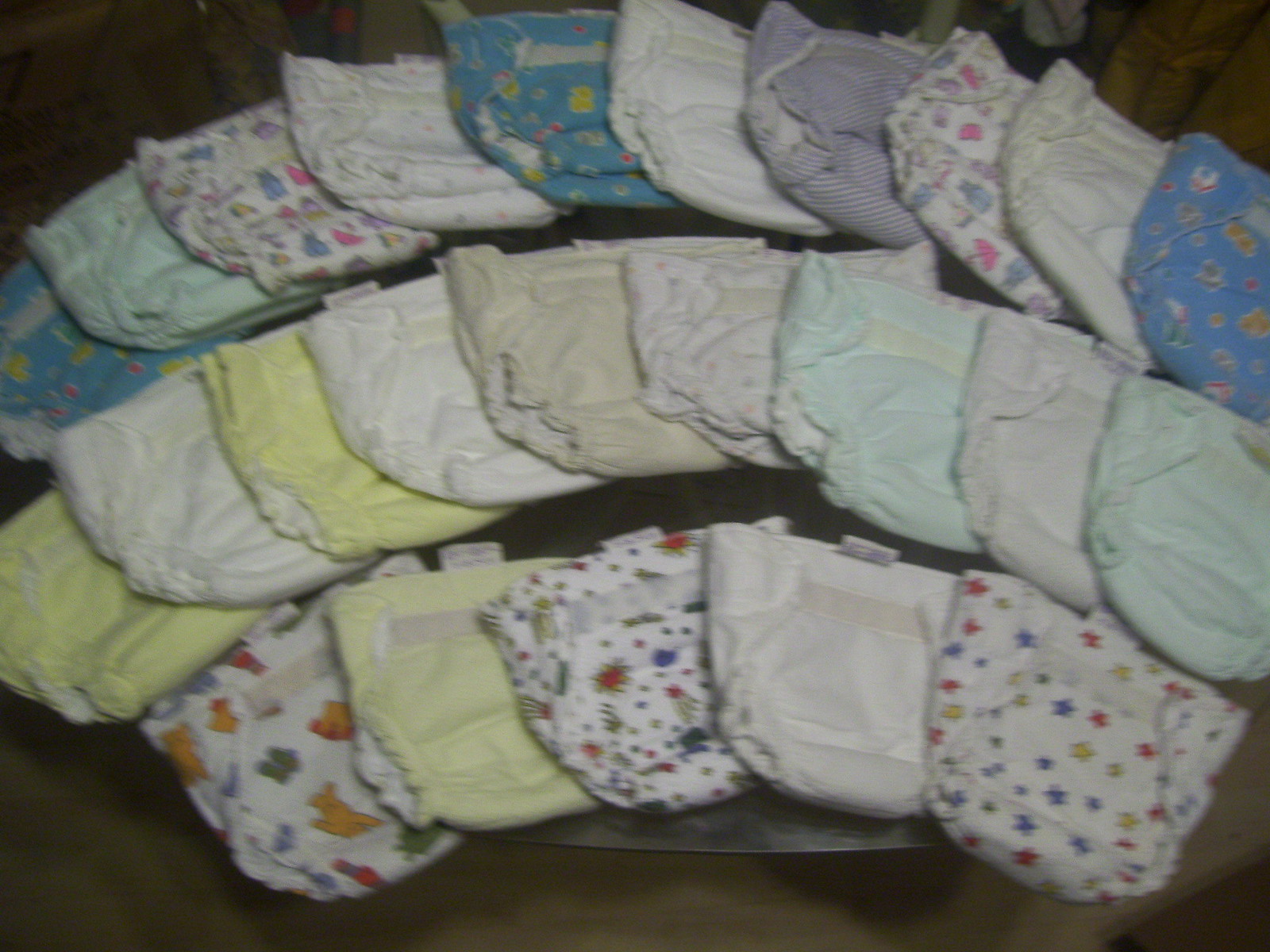In this slightly soft, color photograph, a detailed display of cloth and plastic diapers is arranged artistically atop a glass tabletop set against a dark background. The diapers form three arched rows, each row stacking from left to right and becoming increasingly larger toward the back. The front row features five diapers, including a white one adorned with red, yellow, and blue stars, a yellow one, and one with small artwork in green, dark red, and blue. There are also diapers with depictions of rain jackets, umbrellas, and bear designs. A distinguishable piece is the Winnie the Pooh-themed diaper on the right side, featuring orange and green hues. The second row, slightly larger, and the third, even larger, continue the playful pattern with an assortment of plain white, off-white, light green, blue, and colorful printed diapers. Some diapers exhibit varied patterns like small animals and different colored stars, creating a lively mosaic of colors and prints ranging from purple to light yellow and green. The entire setup is presented on a brown table, although the overall image clarity is a bit fuzzy, slightly obscuring finer details.